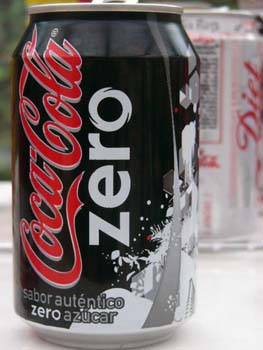This photograph features a can of Coca-Cola Zero prominently displayed on a white table. The can, made of aluminum, sports a sleek black design with "Coca-Cola" written in a dark lipstick red font running vertically up the front. Directly below, the word "zero" is presented in a striking white font, also vertically aligned. At the lower left-hand corner of the can, additional wording can be seen in silver and white, possibly in Spanish. The bottom part of the can features a series of white bubbles, and a silver stripe runs vertically along the right-hand side.

In the background, a can of Diet Coke can be seen, oriented in such a way that only the back label is visible, with the word "diet" partially cut off and running vertically in red. This can is silver in color, typical of Diet Coke, and also made of aluminum. The tabs on both cans appear to be sticking up, although they extend beyond the top edge of the photograph, making it unclear if they are fully open.

Additionally, there is a hint of greenery visible on the left-hand side of the image, adding a subtle touch of natural contrast to the composition.